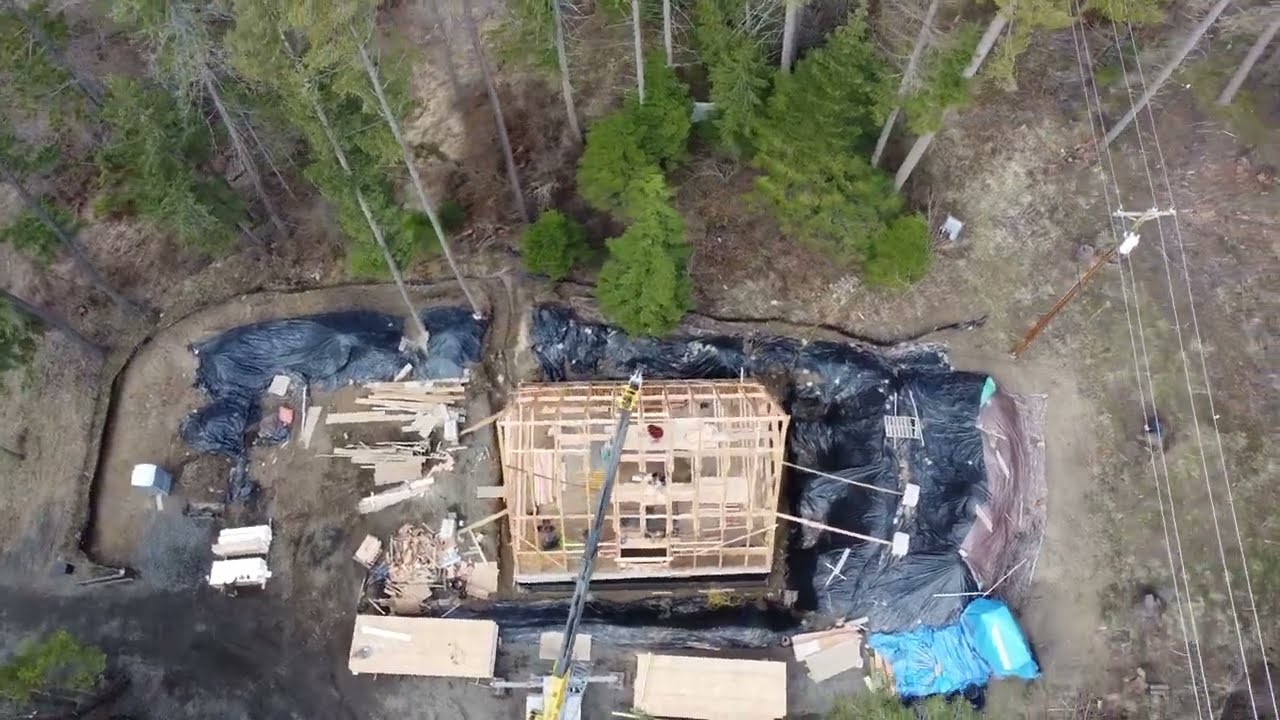The image is a detailed, overhead outdoor photograph of a house under construction, taken during the day. The central focus is the partially built wooden framing of a peaked roof, with a crane positioned in the lower center, lifting additional materials. Surrounding the structure are piles of timber and larger wooden boards. Encircling the construction zone are areas covered with black and blue plastic tarps. The scene is set within a dirt lot bordered by tall green trees that span across the top half of the image, adding a natural backdrop. On the right side, utility lines and a pole run vertically along the image's border, emphasizing the outdoor, semi-rural environment. The image is rich with colors ranging from the earthy browns of the timber and dirt to the greens of the trees, highlighting a sunny, clear day ideal for construction work.